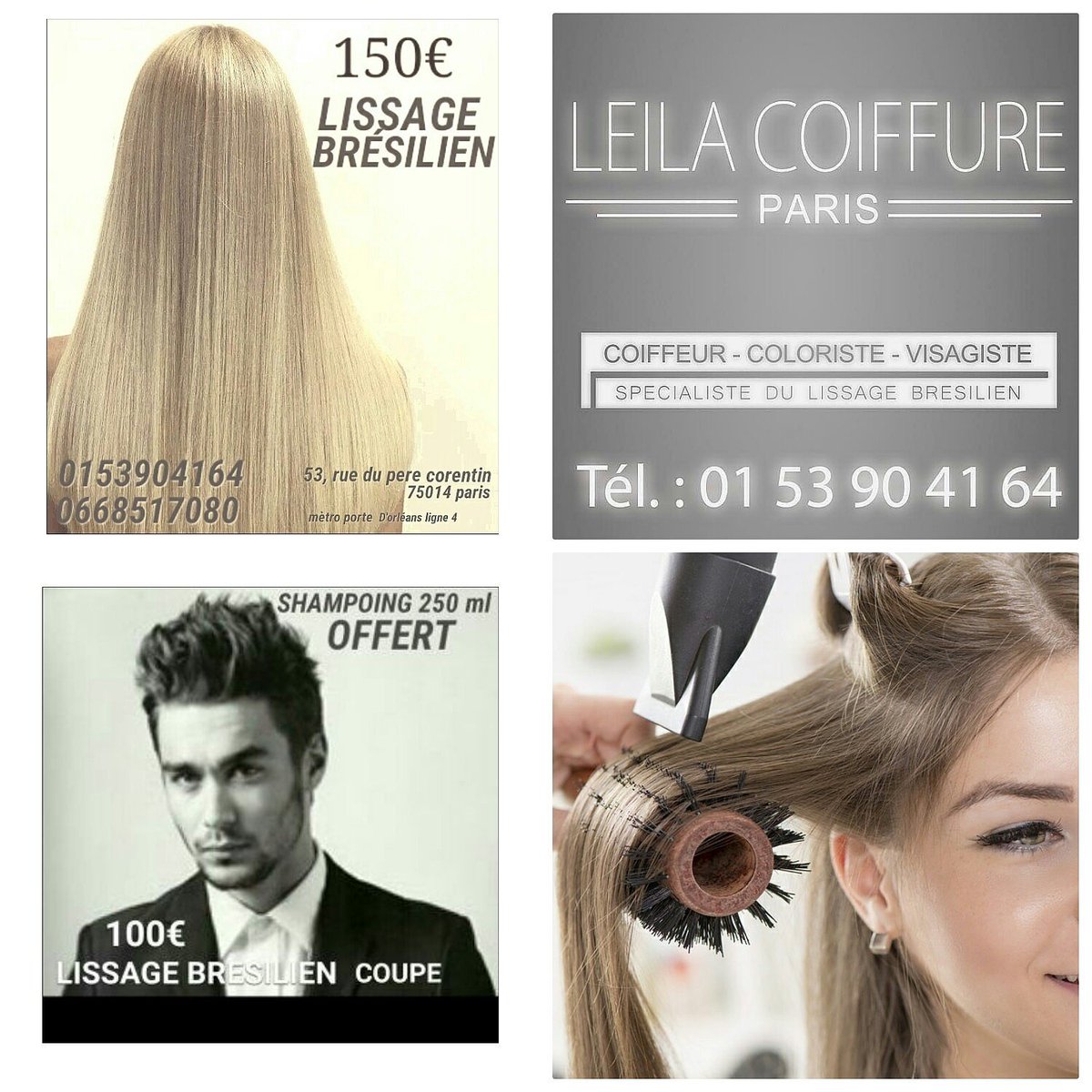This image is a collage-style advertisement for a Parisian hair salon, featuring four distinct sections. The top left section shows the back of a woman’s head with long, beautiful blonde hair, alongside text in French detailing a service priced at €150, mentioning “Lissage Breslien,” and displaying contact information and an address: “53 Rue de Paris, Paris, 75014.” The top right section has a gray background with white text reading “Lila Coiffure, Paris” and continues with detailed service descriptions like “Coiffure Coloriste-Desangiste, Specialist” and another phone number. The bottom left section features a black and white image of a well-dressed man in a suit, with additional service details such as "Shampooing" priced at €250. The bottom right section displays a partial view of a woman’s face with dirty blonde hair being styled using a pink brush and a gray blow dryer, suggesting hair styling services. The entire collage is arranged in a windowpane style, with a mixture of colors including white, yellow, black, gray, brown, and olive, indicative of a sophisticated and professional advertising approach for the salon’s hair treatment and styling services.